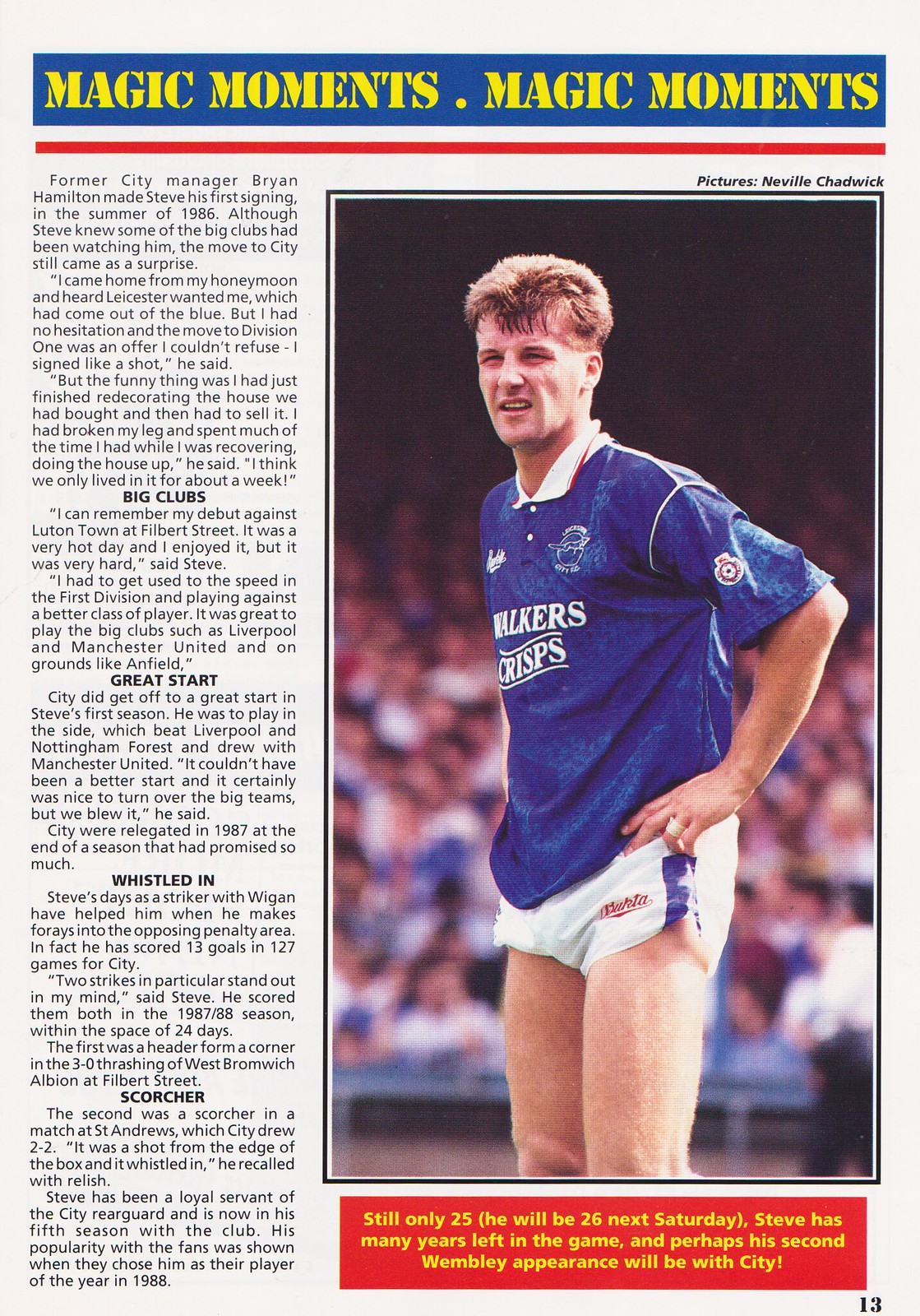This image depicts a scanned page from a sports program or magazine, designed with a blue banner at the top displaying the phrase "Magic Moments, Magic Moments" in a yellow stencil font. Dominating the right side of the page is a full-color, vertical photograph of a contemplative man wearing a blue soccer jersey with the "Walker's Crisps" logo and white shorts, standing with his hands on his hips amidst a crowded stadium. The man, identified as Steve, has short blonde hair and is described as being on the verge of turning 26 next Saturday. A red text box at the bottom states, "Still only 25. He'll be 26 next Saturday. Steve has many years left in the game and perhaps his second Wembley appearance will be with City." Along the left side of the image is a large column of text in black against a white background, detailing Steve's biography and career. It describes how former City manager Brian Hamilton made Steve his first signing in the summer of 1986, despite some big clubs showing interest. The text includes sections labeled “great start,” “whistled in,” and “scorcher.” This comprehensive presentation provides a detailed look at Steve's background and achievements.